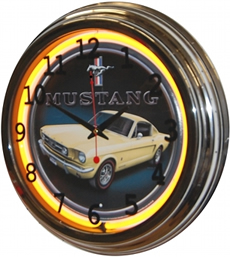The image depicts a vintage clock with an intricate design centered around a classic automotive theme. The clock's face prominently features a yellow 1960s Shelby Mustang. Above the car, the word "Mustang" is inscribed in bold letters, with the iconic Mustang emblem placed just below the 12 o'clock marker. Surrounding the car are large, black numerals in a traditional clock layout, running from 1 to 12.

Encircling the face of the clock is a vivid yellow neon light, which stands out against a sleek black border. Adjacent to this border is a band of silver chrome, resembling the rim of a car wheel, lending a polished, automotive finish to the overall design. The hands of the clock indicate a time of 1:50:59.

At the bottom of the image, the website "www.mytrendyphone.co.uk" is subtly displayed, suggesting the likely source or retailer of this retro-styled Mustang clock.